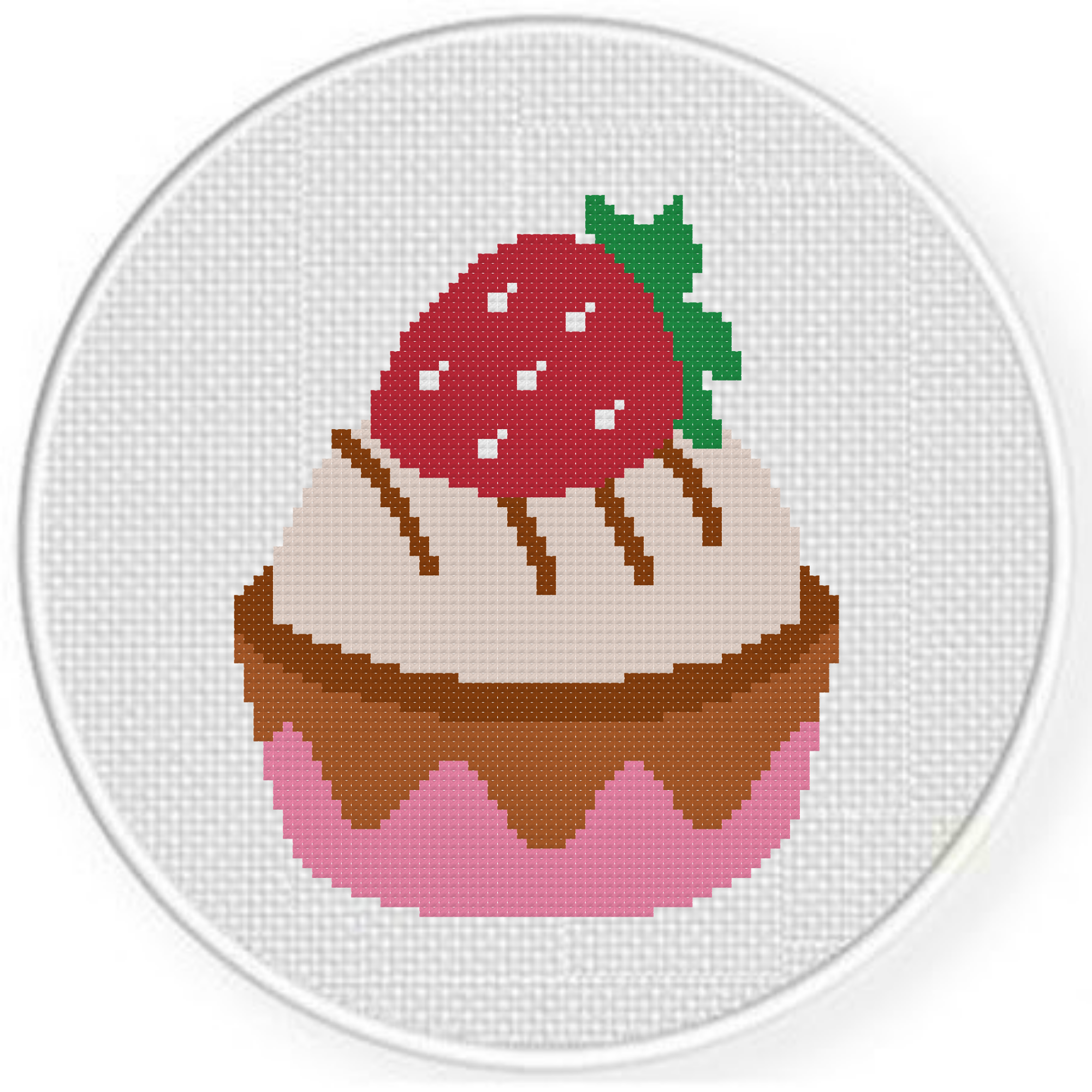This detailed and vibrant image showcases a round embroidery hoop featuring a meticulously crafted cross-stitch pattern. The fabric inside the embroidery hoop is stark white, creating a clean backdrop that emphasizes the colorful central subject. The central design is a delectable cupcake adorned with intricate details: a base in shades of pink, topped with layers of light and dark brown that suggest rich chocolate. Crowning the cupcake is a creamy vanilla scoop, presumably ice cream, adorned with a sprinkling of dark brown chocolate accents. Atop this sits a vivid red strawberry, complete with a green calyx, its white seeds glistening as if reflecting light. The image, captured in a square format, ensures focus on the carefully embroidered details, suggesting a commercial use, possibly illustrating a pattern available for purchase. This photographic representation highlights the artistry involved in creating this hand-stitched piece, emphasizing its realism and appeal to those interested in the craft of embroidery.